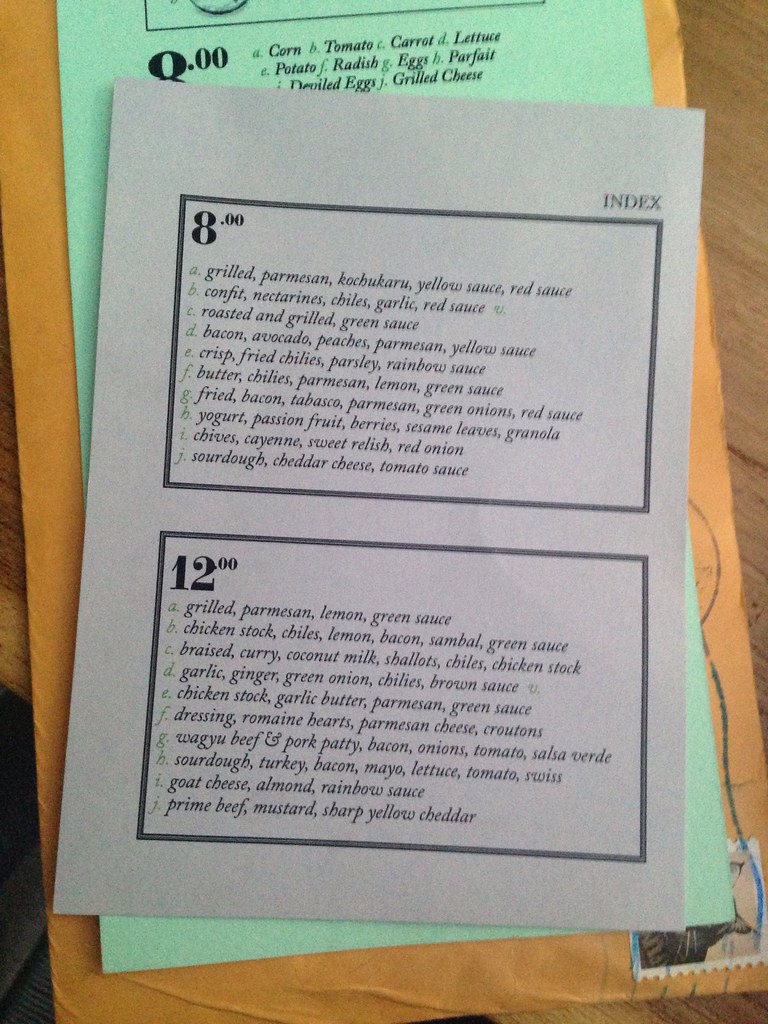A simple yet intriguing menu layout is depicted on a plain gray sheet of paper. The menu is divided into two sections, each outlined with black frames positioned in the upper right corner, and the label "index" faintly printed on it. Notably, the gray sheet lacks any prominent heading or logo.

In the upper left of the first box, the price $8 is highlighted, followed by a long list of diverse culinary items such as Grilled Parmesan, Kochukaru, yellow sauce, red sauce, confit, nectarines, chilies, garlic, roasted and grilled green sauce, bacon, avocado, peaches, Parmesan, crisps, fried chilies, parsley, rainbow sauce, butter, lemon green sauce, fried bacon, Tabasco, green onions, yogurt, passion fruit, berries, sesame leaves, granola, chives, cayenne, sweet radish, red onion, sourdough, cheddar cheese, and tomato sauce.

The box below it is similarly structured but lists $12 items. These include Grilled Parmesan, lemon green sauce, chicken stock, chilies, lemon, bacon, sambal green sauce, braised curry, coconut milk, shallots, garlic, ginger, green onion, brown sauce, butter, dressing, romaine hearts, Parmesan cheese, croutons, Wagyu beef and pork patty, bacon, onions, tomato, salsa verde, sourdough, turkey, bacon, mayo, lettuce, tomato, Swiss, goat cheese, almond, and prime beef with sharp yellow cheddar.

Below this gray sheet, an edge of a longer green menu peeks out, skewed slightly to the right. The top part of this green sheet displays an $8 price, with visible items such as corn, tomato, carrot, lettuce, potato, radish, eggs, parfait, deviled eggs, and grilled cheese. A small black box above this list contains an indistinct image.

Both sheets rest atop a manila envelope, which is oriented vertically. Notably, in the bottom right of the image, partially covered by the green menu sheet, there is a cat-themed postage stamp with a postal mark indicating the envelope has been previously mailed.